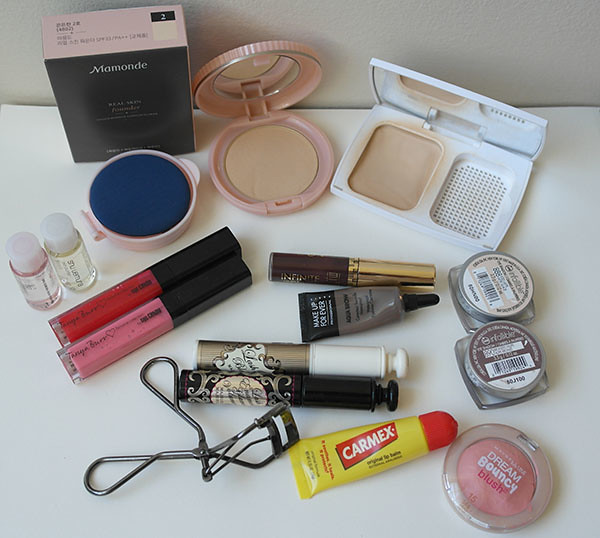This image showcases an elegant array of makeup and toiletries meticulously arranged on a white countertop, with an off-white backdrop likely cast into shadow. 

In the upper left corner, there's a striking black box with pink trim inscribed with the brand name "MAMANDE," although smaller text beneath is too indistinct to decipher. Adjacent to this box lies a pink circular compact housing a blue sponge. To its right, another pinkish compact powder joins the display.

At the top right, there is a white rectangular container whose contents could be makeup, blush, or bronzer, though identification is uncertain. Directly below, two round, semi-clear containers sit without easily discernible labels.

In the bottom right corner stands a clear round container labeled "Dream Bouncy Blush," boasting a pinkish hue. Accompanying it is a recognizable tube of Carmex, an eyelash curler, and a diverse assortment of items in the middle. These include multiple lip gloss tubes in shades of pink – ranging from pale to dark – and several other tubes with indeterminable labels.

On the far left, the arrangement is completed by two small, clear round bottles, the contents of which remain unreadable due to their size. The collective presentation forms a visually pleasing and well-organized collection of beauty products.